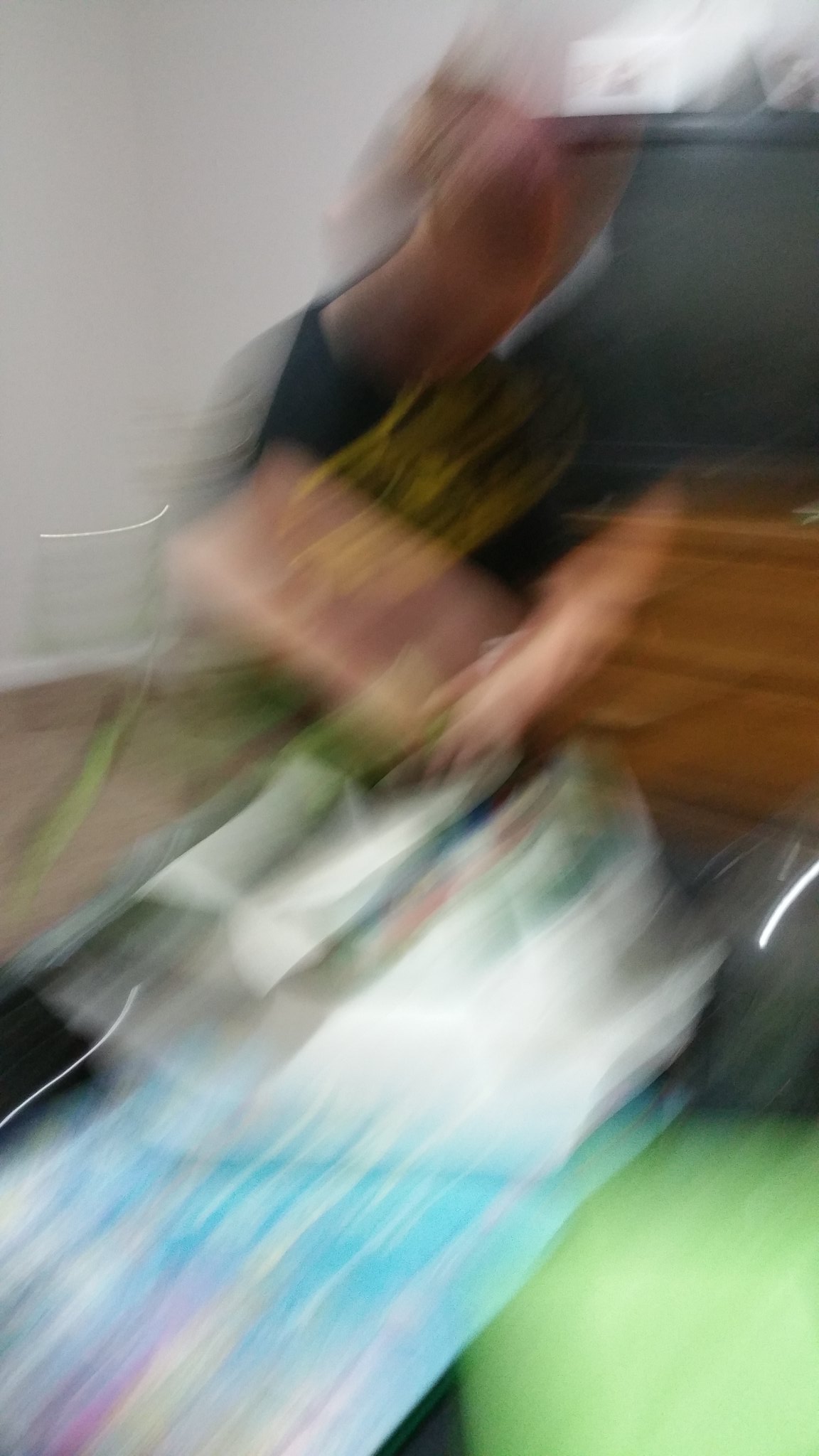In this very blurred photograph, a woman with blondish hair is captured sitting against a white wall. She is wearing a dark shirt adorned with yellow lettering. The woman's figure and movements are indistinct due to the blur, but she seems to be holding or possibly opening a rectangular-shaped item. Underneath this item, a vibrant mix of colors - blue, white, green, and yellow - can be spotted. 

The setting includes a notable older style television, positioned on an oak-colored chest of drawers. Atop the television, a conspicuous white box is placed. In the bottom right corner of the image, there is a green blob, which could either be an item captured in the frame or the photographer's thumb partially covering the lens. Despite the blur, the scene conveys a sense of activity, possibly suggesting the woman is in the midst of unwrapping a gift.